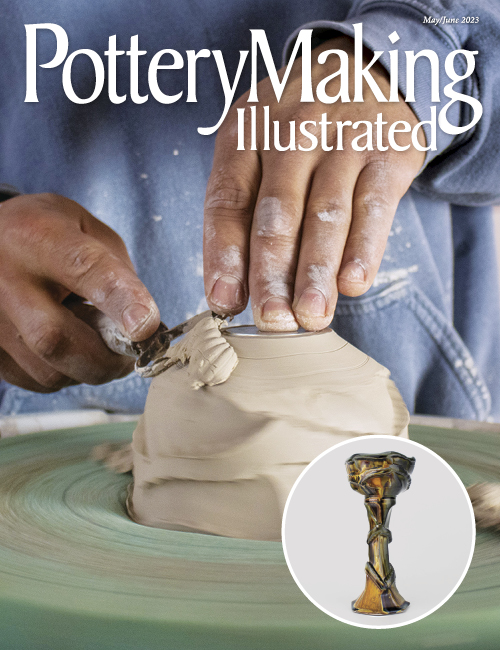The cover image of the May-June 2023 issue of *Pottery Making Illustrated* prominently displays the finely detailed process of pottery crafting. The title "Pottery Making Illustrated" is emblazoned in bold white letters at the top, and "May-June 2023" is noted in smaller white text in the top right corner. The central image features a pair of hands, dark-skinned and skillful, artfully shaping a piece of wet light brown clay on a spinning light green potter's wheel. The left hand is pressed firmly upon the clay, guiding its form, while the right hand skillfully maneuvers a metal tool, shaving thin curls of clay off the developing shape. Subtle yet prominent, a blue jacket partially covers the upper part of the image, hinting at the potter's attire. In the lower right corner of the cover, a small picture-in-picture inset showcases an intricate, copper-colored chalice within a gray circle, suggesting a finished piece that may be a goal for the potter's current work.